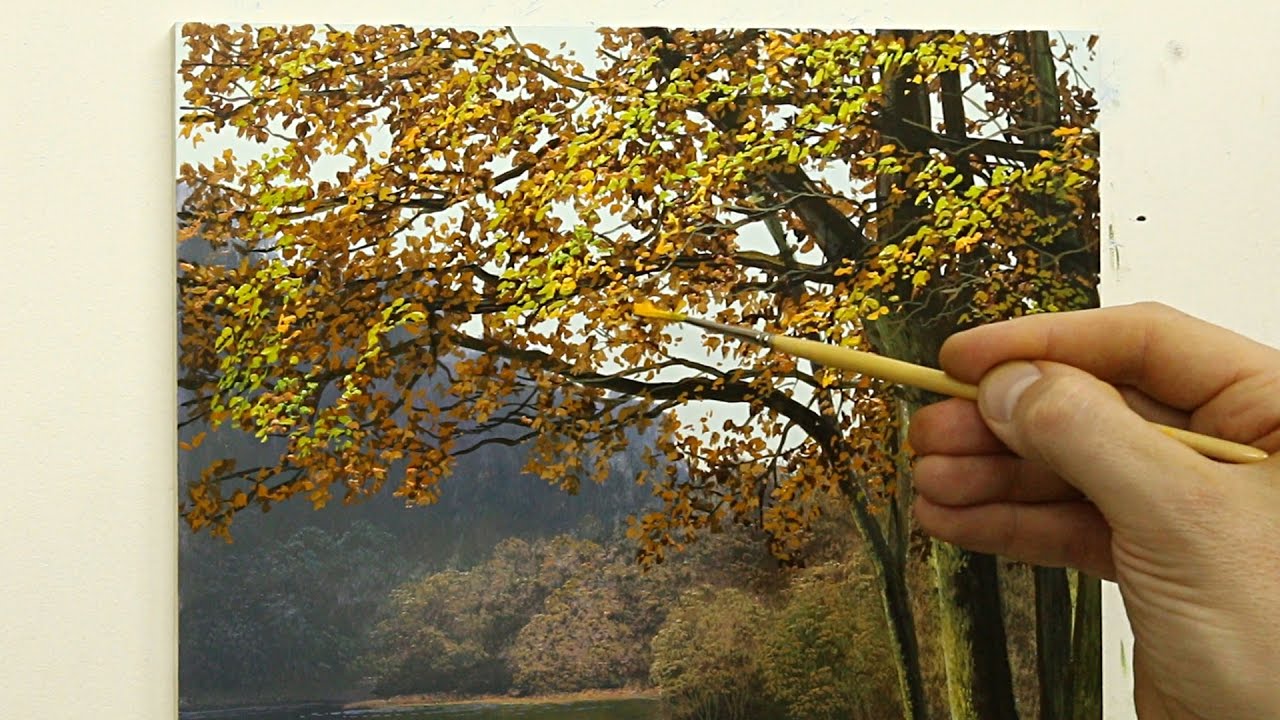In this photograph, a nearly complete rectangular painting is centered prominently against a light cream wall backdrop. The painting is a vivid autumn scene featuring a tree with an array of yellow and green leaves. Behind this main tree, additional trees and a mountain range can be seen under a clear sky. A Caucasian hand is visible on the left side of the image, delicately holding a small paintbrush. The paintbrush, with a cream-colored handle and silver metallic ferrule, has its tip currently dipped in yellow paint. The artist is meticulously applying the yellow paint to the leaves of the foreground tree, demonstrating their impressive skill in rendering lifelike details. The immersive quality of the painting and the profound realism of the tree attest to the artist's exceptional talent and precision.